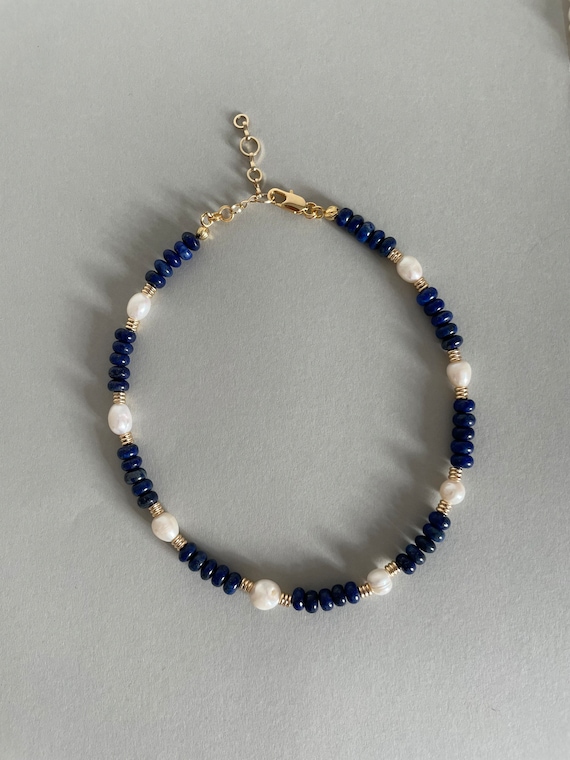The image features a piece of jewelry, likely a bracelet, displayed against a uniform pale blue background. The bracelet's design consists of a repeating pattern of five blue beads, interspersed with a white pearl-like bead. The blue beads are divided into sections by gold-tone beads, which create a striking aesthetic contrast. The clasp of the bracelet is also gold-tone and includes a small adjustable chain for sizing. The detailed pattern unfolds as follows: five blue beads, one white pearl, and then another set of five blue beads, repeating all around the bracelet. The central arrangement includes a sequence of five blue beads, one white pearl, two white pearls next to each other, and another set of five blue beads, highlighting the intricate design.